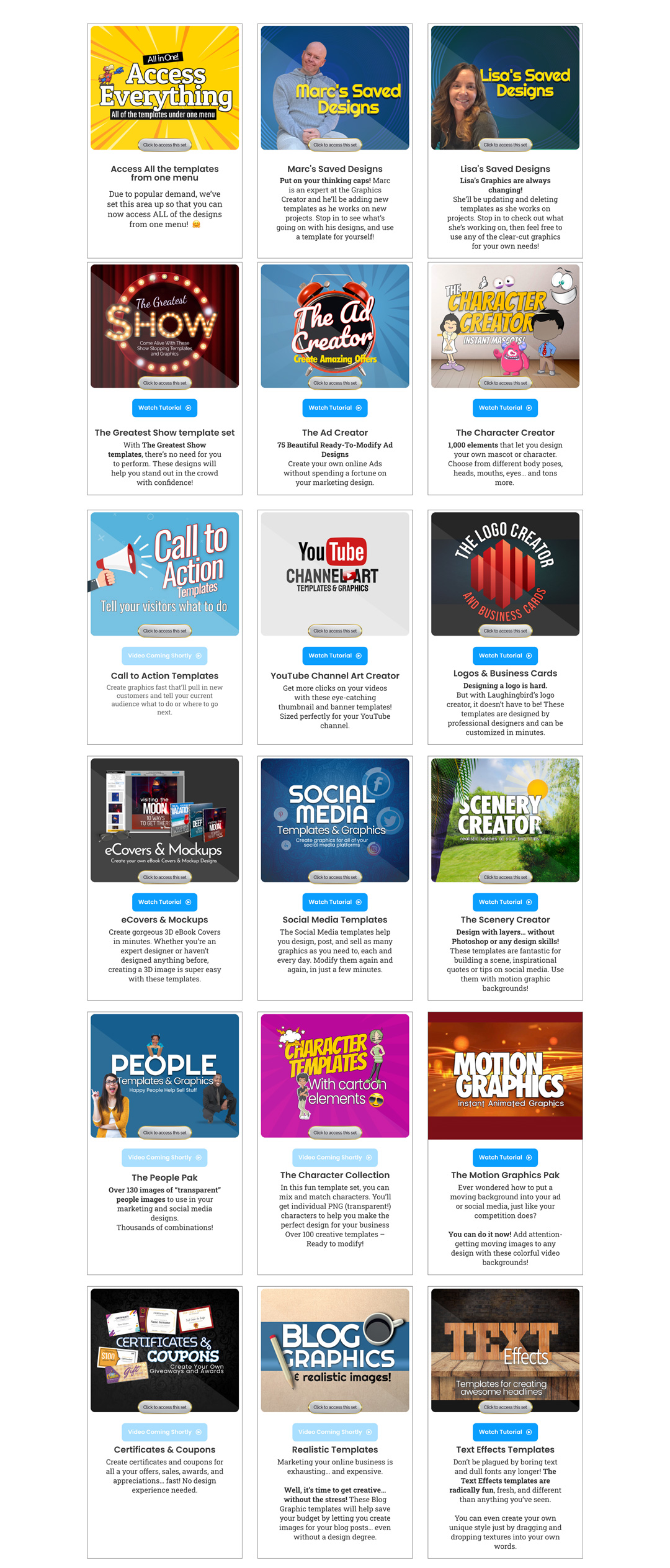The image displays a grid-like interface reminiscent of a smart TV guide but centered around creative design tools and resources. Organized into a series of rectangular blocks resembling channels, each block represents a different design tool or resource. The titles of these blocks include "Access Everything," "Mark's Saved Designs," "Lisa's Saved Designs," "The Something Show," "The Ad Creator," "The Character Creator," "Call to Action," "YouTube Channel Art," "The Logo Creator," "E-Something and Mockups," "Social Media," "Scenery Creator," "People," "Character Templates," "Motion Graphics," "Certificates and Coupons," "Blog Graphics," and "Text Effects." Beneath each title and corresponding image, there is a brief descriptive blurb that is unfortunately unreadable due to the image's pixel density. Despite the unclear text, the visual layout clearly aims to facilitate various creative projects, ranging from social media graphics and YouTube channel art to motion graphics and blog visuals.